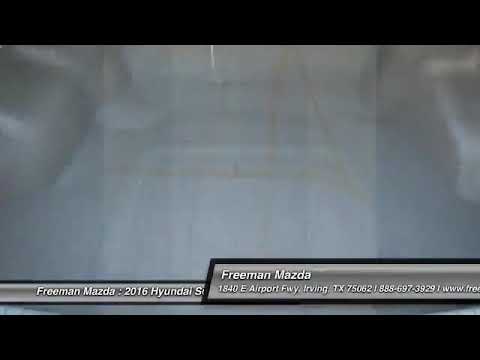The image appears to be a still from a video with a gray background dominated by indistinct shapes, faint lines, and a checkerboard pattern of lighter and darker gray areas. Along the bottom of the image, there are two horizontal rectangular text boxes with black outlines. The first, smaller gray box on the left features white text that reads "Freeman Mazda: 2016 Hyundai S," but part of it is obscured by the second, larger gray box. This larger box, positioned diagonally over the first, also has a black outline and contains the text "Freeman Mazda" in bold, followed by "1840 East Airport Freeway, Irving, Texas 75062" in smaller letters. There is also a phone number, 1-888-697-3829, and the beginning of a web address, "www.free," which is cut off by the image's right edge. The top and bottom edges of the image are bordered by thick black lines. An element in the middle resembles a vertical white rectangle overlain by a formation resembling the letter ‘A’ made out of yellow diagonal and horizontal lines, suggesting it could be a reflection or some sort of background object. Overall, despite the unclarity of the central area, the text clearly indicates it is an advertisement for Freeman Mazda, featuring a specific vehicle model and contact information.